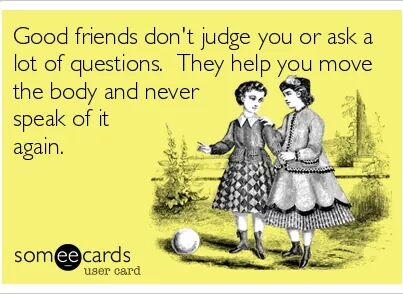This image features a Sun-Yi card with a yellow background and black font. Across the top, the card humorously states, "Good friends don't judge you or ask a lot of questions. They help you move the body and never speak of it again." On the right side of the card, there's an old-fashioned drawing of two young girls dressed in 1800s attire, complete with long-sleeved dresses and black boots. One girl, possibly wearing a bonnet, points into the distance, while the other looks on. They are depicted standing outside in a wooded area with trees and possibly a body of water in the background. In front of them on the ground, there appears to be an egg. In the bottom left-hand corner, it reads "Sun-Yi cards, a user card."